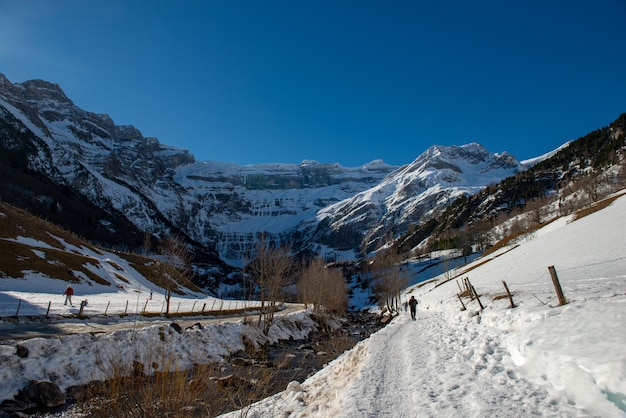A pristine, snow-covered mountain landscape stretches into a clear blue sky, with no clouds to obscure the view. In the foreground, to the left, a skier in a red jacket navigates down the slopes, while on the right, a person dressed in black walks alongside some brown poles. This right-side figure is near a ravine flanked by barren brown trees. A narrow, black asphalt walkway, almost hidden but still visible, cuts through the snow-covered terrain. Within the ravine, a stream can be seen snaking through rocks, complimenting the expanse of white snow with its fluid motion. Farther up the valley, small, leafless trees punctuate the otherwise snow-draped landscape. In the image's backdrop, impressive and towering mountains, their peaks dusted with snow, rise sharply into the sky. The scene is a blend of white snow, brownish vegetation, black asphalt, and the vibrant blue sky, capturing the serene and majestic essence of the frozen wilderness.